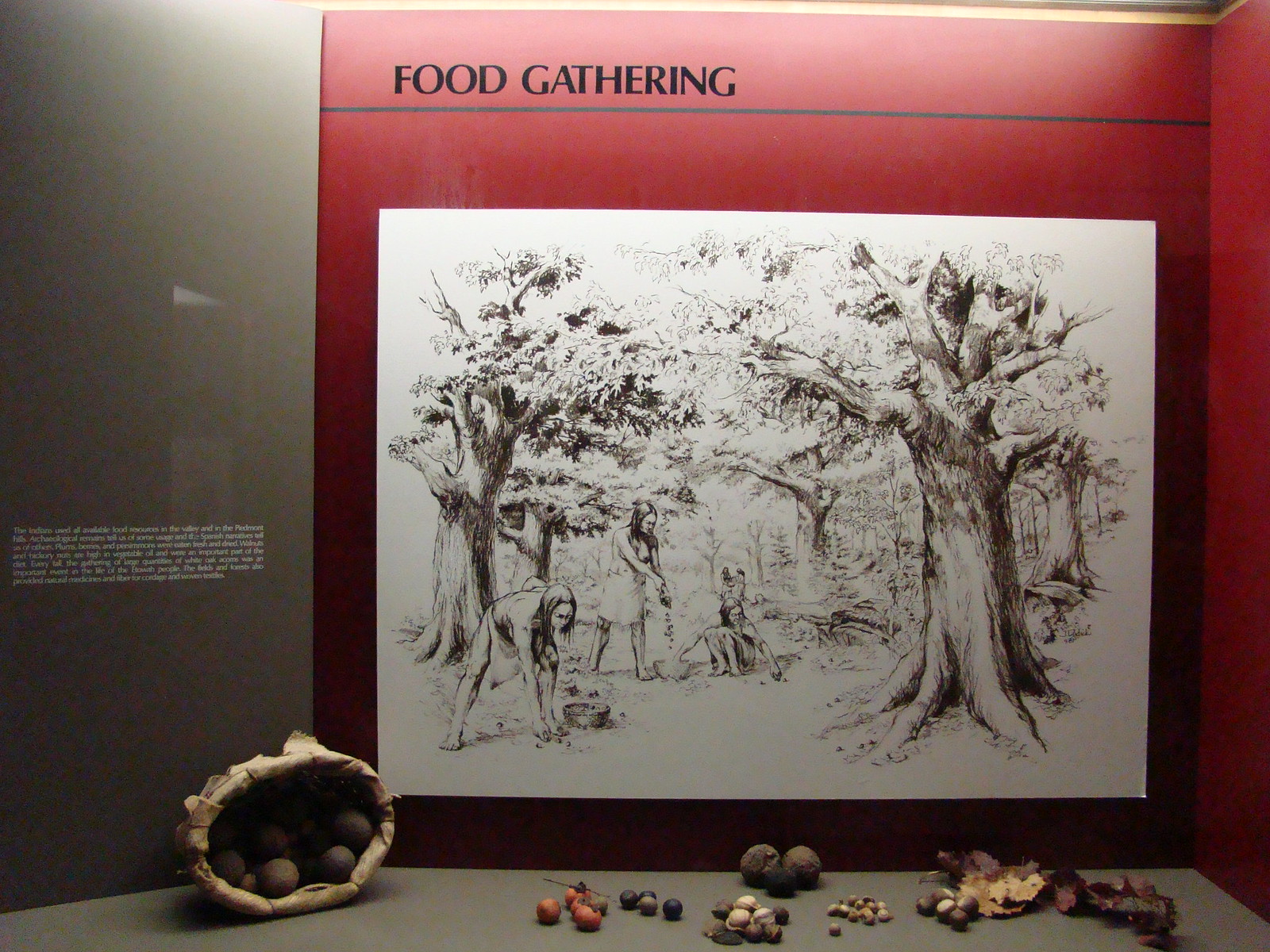The black and white pencil sketch at the center of this museum exhibit, entitled "Food Gathering," depicts a serene woodland scene where several primitive human figures are engaged in gathering activities. At the heart of the artwork, a girl stands amidst the trees, while another girl sits on the ground, and a third bends over to pick something up. The detailed sketch is framed in a vibrant red border, with the title "Food Gathering" emblazoned in black letters at the top. Adjacent to the red border, a contrasting gray background contains a descriptive paragraph in white letters. In the foreground, the exhibit features a realistically crafted basket filled with mock seeds or nuts, providing tangible context to the drawing and enhancing the historical narrative of human subsistence practices.